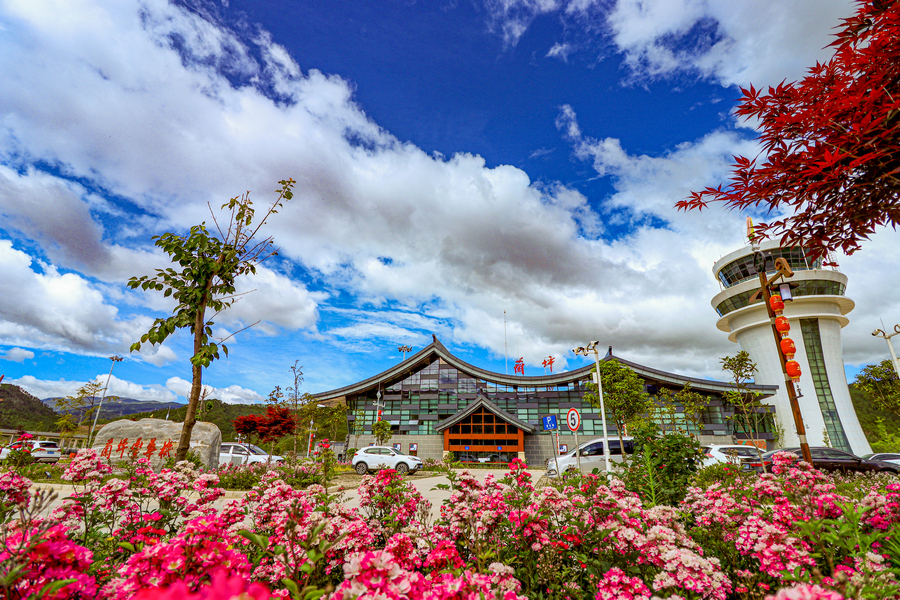This image captures a striking scene in what appears to be a foreign country, potentially Japan. Dominating the background is a modern pagoda-style building with distinctive curved and peaked roofs, reminiscent of traditional Japanese architecture. The structure features a façade almost entirely composed of glass windows, underpinned by a brick foundation, and there's a white tower at one end. A red entryway adds a pop of color, while lanterns on posts are scattered around the property, infusing a sense of cultural charm.

In the foreground, an immaculately maintained garden bursts with vibrant pink and white flowers, spanning the bottom fifth of the photograph. Amidst this floral display stands a striking Japanese maple tree with vivid red leaves, positioned to the right. To the left and slightly behind the flowers, a large rock marked with red script—illegible to the observer—suggests it may serve as a sign or landmark for the building.

There are several cars parked in a lot in front of the building, predominantly white with a couple of other colors mixed in. The backdrop features gentle hills, enhancing the scenic quality of the location. Overhead, the sky transitions from a deep to a lighter blue, adorned with scattered clouds, adding a serene and picturesque aspect to the overall composition.